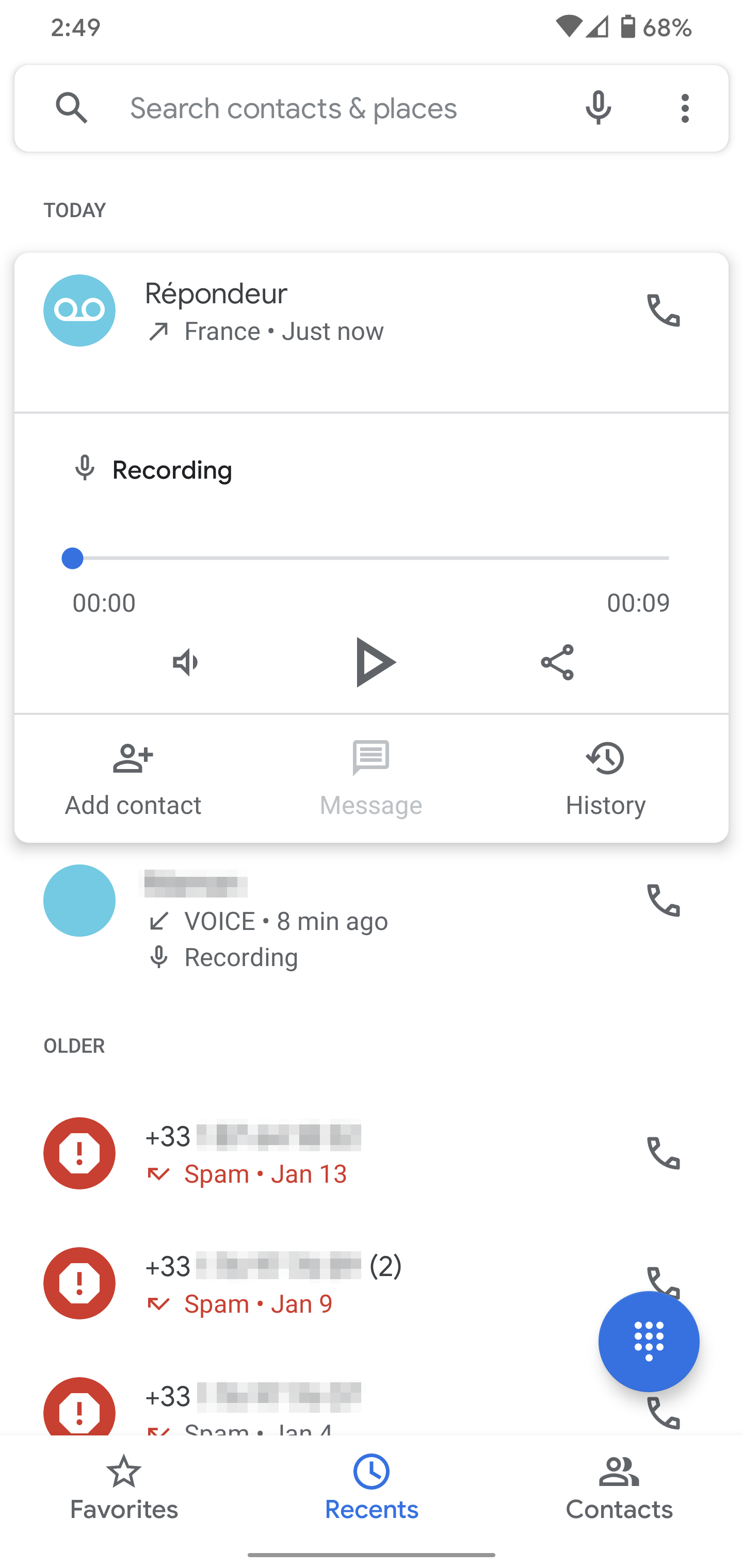### Descriptive Caption:

This screenshot depicts the user interface of a smartphone, captured at 2:49 PM. It shows several key details about the phone's status, including Wi-Fi access, low cellular signal, and a 68% battery charge. At the top of the screen, there is a search bar labeled "Search Contacts and Places," accompanied by a microphone button and a three-dot menu icon for additional options. Directly below, a white triangle indicates the current section "Today," specifying the location "Les Pondus, France" with a "just now" timestamp.

The main feature of the screenshot is a recording interface that includes a recording symbol, a timeline for tracking the audio, and buttons for "Go," "Share," and "Volume." There’s also an "Add Contact" option, followed by sections labeled "Message" and "History." 

A blue oval marked "Voice, 8 minutes ago" appears underneath, indicating another audio recording feature with a microphone icon beside it. Below this, the user has three entries marked with red exclamation points inside red circles. These entries list phone numbers starting with "+33," all identified as "Spam," and are dated January 13th, January 9th, and January 4th respectively. Each entry includes a telephone icon beside it.

At the very bottom of the screen, a footer contains navigation tabs labeled "Favorites," "Recents," and "Contacts," all set against a clean, white background.